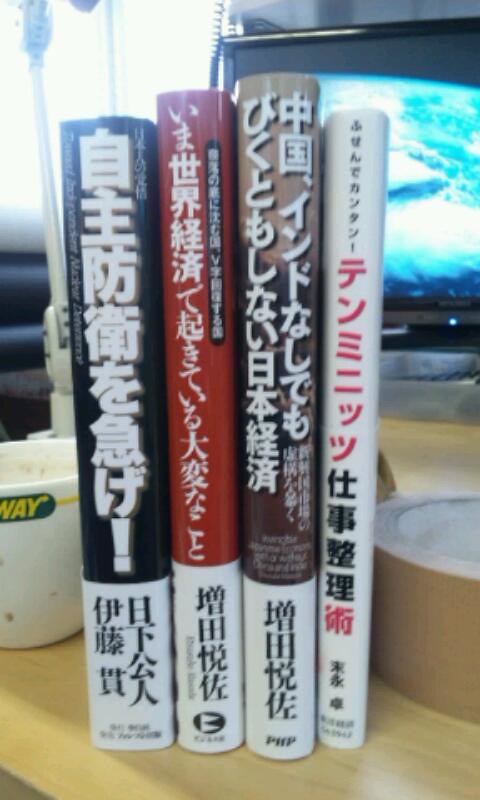In the image, four books with East Asian characters, possibly Japanese, are standing side-by-side on a desk, showcasing their multicolored spines. The spines exhibit varied color schemes: one is black with white and red text, another is brown with white and black text, the third is red with white and black text, and the fourth is white with white and black writing, possibly with a blue strip. To the left of the books is a small Subway cup, easily identifiable by its partial "way" text and signature yellow and green branding. A roll of masking tape is positioned to the right of the books. Further back on the desk sits a computer displaying an Earth wallpaper with windows in the background letting in dim, gloomy daylight. The room is softly lit by the muted sunlight filtering through the windows.